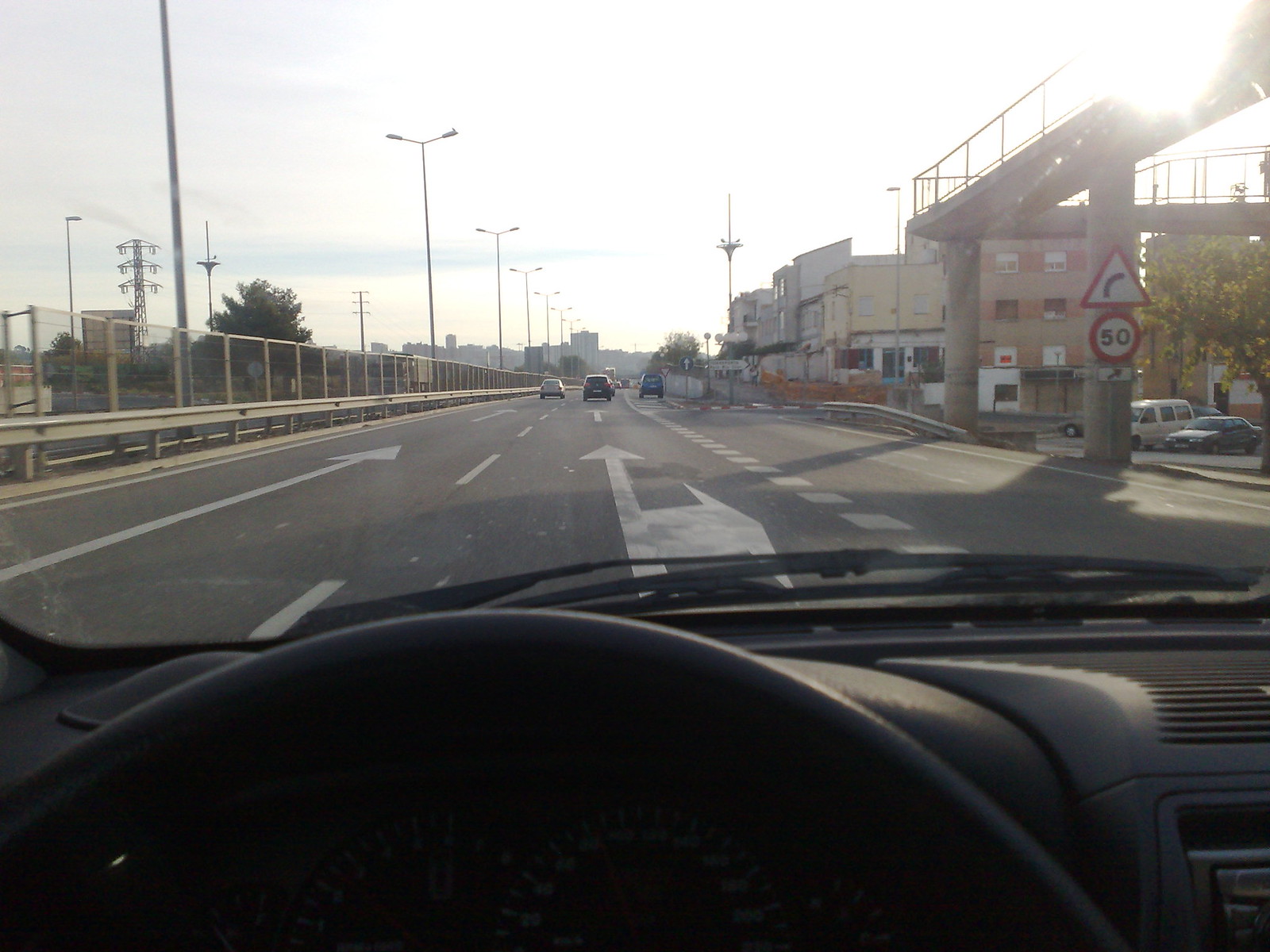This color photograph captures the view through the windshield of a car as it travels down a multi-lane urban road, combining three detailed descriptions. The dashboard, which is black, frames the image, while the solid-looking steering wheel sits prominently in the foreground. The road ahead features multiple white arrows: two pointing forward and one directing traffic to the right. To the left, a metal chain-link fence secures the area behind a guardrail, beyond which you can see streetlights, electric poles, and a satellite or electrical tower. The streetlights along the left have one lamp each, while those nearer the middle have dual lamps extending from either side of the poles. To the right, a series of rectangular buildings with small square windows line the street, and a high, cement-supported walkway or bridge stands over a line of parked cars. Prominent street signs are attached to one of the cement supports – a triangular white sign with a red border and an arch-like black symbol, positioned above a circular sign marked '50,' also white with a red border.